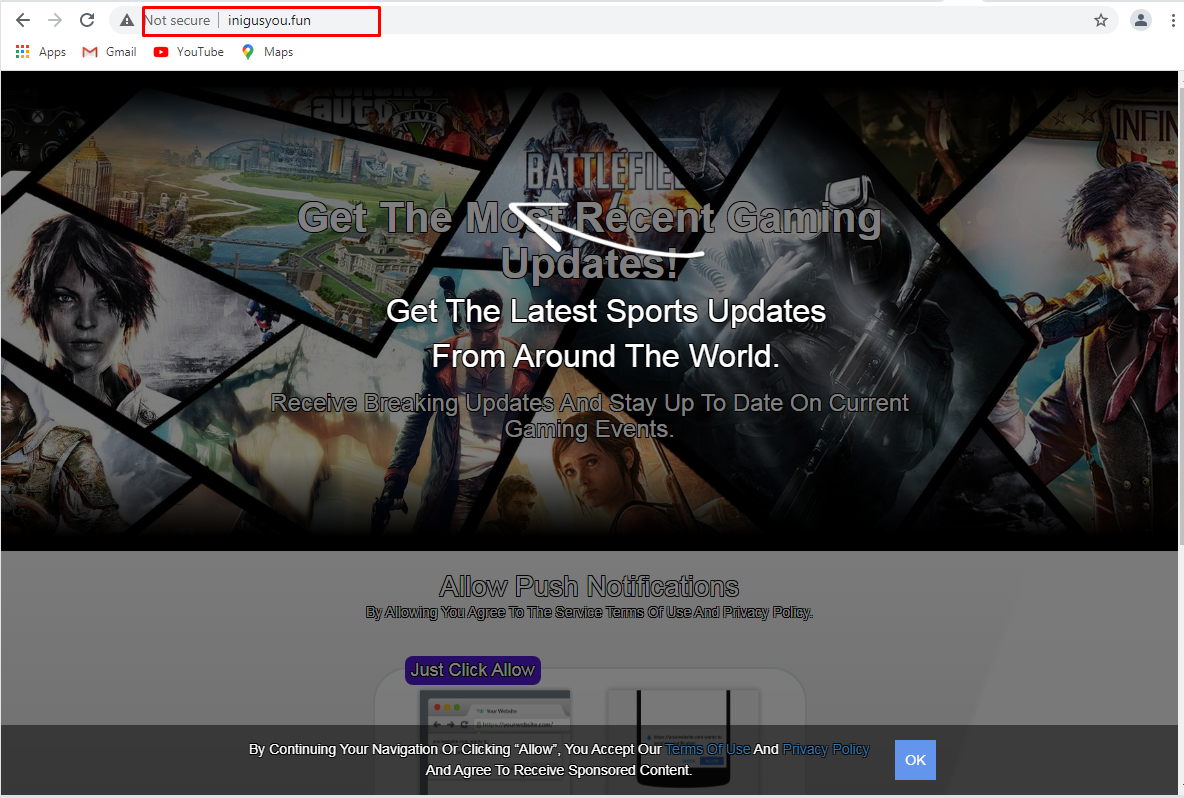A screenshot of a website is captured in this image. The address bar at the top indicates the URL "inigosu.fun" and shows a "Not Secure" warning. In the upper right corner, there's a circular icon featuring a silhouette of a person's head and shoulders. Below this, the options "Apps," "Gmail," a YouTube logo followed by "YouTube," and "Maps" are listed.

The main portion of the screen displays a large, dark, and overcast image that seems to feature various video game elements. This image includes a female video game character posing as a fighter, an animated cityscape likely to be a video game setting, a man with a sword strapped to his back, and another man holding a gun.

In the middle of the image, there is prominent text that reads "Battlefield" and "Get the most recent gaming updates," accompanied by a white arrow pointing left. Further text below offers instructions: "Get the latest sports updates from around the world. Receive breaking updates and stay up to date on current gaming events." 

The website prompts users to allow push notifications, stating: "By allowing, you agree to the service terms of use and privacy policy. By continuing your navigation or clicking 'Allow,' you accept our terms of use and privacy policy and agree to receive sponsored content." An "OK" button is visible beside this text.